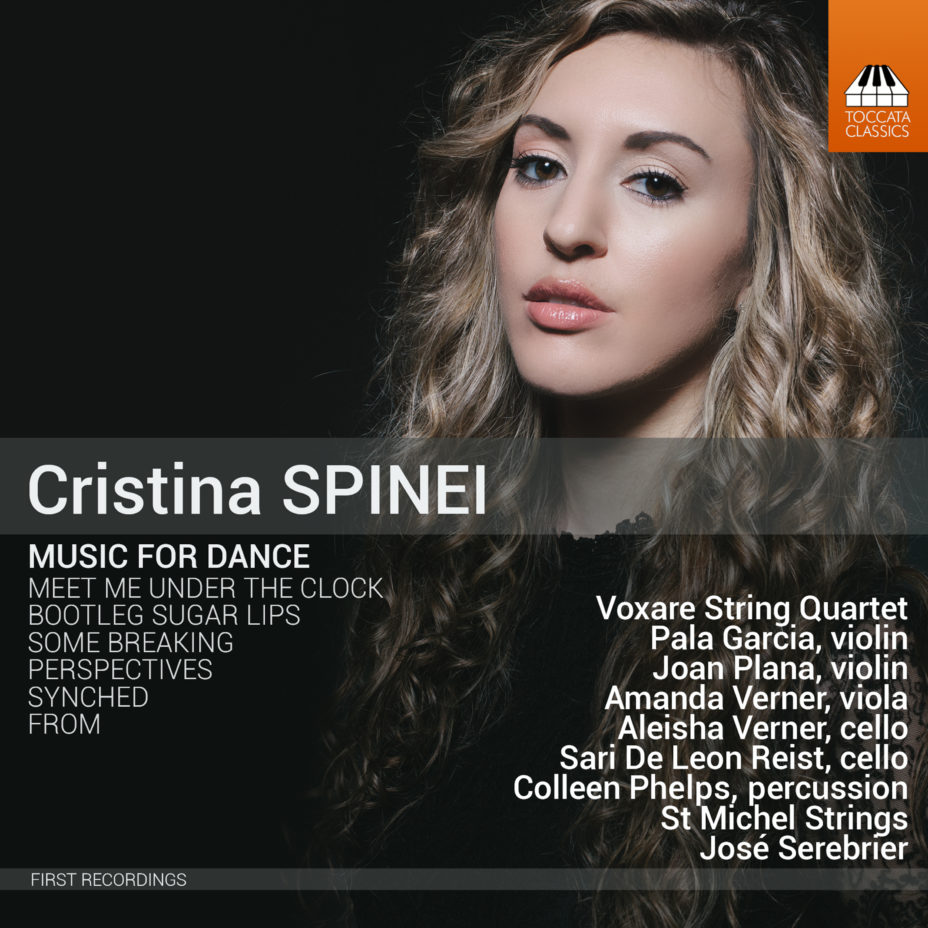The given image is a graphical poster resembling the cover of an album titled "Music for Dance" by Christina Spinei. On the right side of the image, there is a black-and-white photograph of a woman with long wavy blonde hair, dark eyes, dark eyebrows, and pink lips, who is looking directly at the camera with her head slightly tilted to the left. In the upper right corner, there is an orange rectangle featuring the Toccata Classics logo, which resembles piano keys. 

The central part of the image features text from top to bottom that includes the artist's name "Christina Spinei," spelled out as S-P-I-N-E-I, followed by the album's title "Music for Dance." Beneath this are the track titles: "Meet Me Under the Clock," "Bootleg Sugar Lips," "Some Breaking Perspectives Synced From." 

Towards the right side of the image, overlaid on the photograph of the woman, are the names of contributors to the album: Oxare String Quartet, Paula Garcia (Violin), Joan Plana (Violin), Amanda Werner (Viola), Alicia Werner (Cello), Sari D. Leon (Raised Cello), Colleen Phelps (Percussion), St. Michael Strings, and Jose Cerebrier. Finally, at the bottom left corner of the image, the text "First Recordings" is displayed.